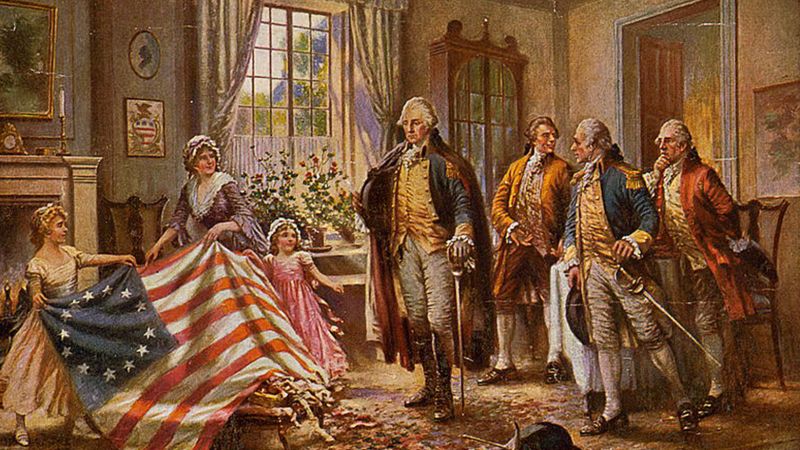This painting, set in an elegantly decorated room around the time of America's founding, depicts Betsy Ross presenting her early design of the American flag to George Washington. Betsy Ross stands between two young girls, all three clad in long dresses and bonnets; the girl on the left in a light yellow dress with heels, the girl on the right in a pink dress. Betsy dons a purple and white conservative dress with a white bonnet. The trio holds an American flag featuring thirteen stars: the girl on the left grips the left edge, Betsy the middle, and the girl on the right the right edge.

Central to the scene is George Washington, standing in a military outfit—a dark blue coat, rich yellow shirt, khaki pants, and high boots—holding a sword pointed down. He is flanked by three men, one in civilian attire—a brown suit with ruffles and white stockings—and two in military garb akin to Washington's. Everyone in the painting is white.

The background showcases a white fireplace with a mantelpiece adorned with an antique clock and a candle in a gold holder, above which hangs an indistinct framed picture. To the right of the scene is a large hutch possibly for china, and a doorway leading to another room. There are multiple wall paintings, a window with green curtains and brown wooden panes displaying trees outside, and a table by the window adorned with orange and yellow flowers. The room, filled with period-appropriate furnishings and decor, provides a refined setting that emphasizes the historical significance of the moment, as four revered American Founding Fathers admire the nascent symbol of their new nation. The palette includes colors such as black, white, gray, brown, yellow, blue, pink, and green, enhancing the historic and patriotic atmosphere of the artwork.